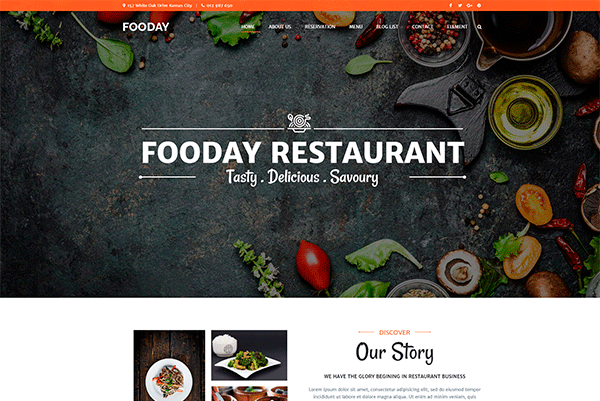The image is a screenshot of a website for Food Day Restaurant. The background features an array of vibrant ingredients, such as sliced tomatoes, red chili peppers, basil, mint leaves, a bowl of olive oil, and a bowl of peppercorns, all suggesting a focus on fresh, quality components. An orange stripe at the top of the page contains the restaurant's contact number, address, and links to its social media platforms, which include Facebook, Twitter, Instagram, and Google+.

Centered prominently on the page is the restaurant's name, "Food Day Restaurant," written in elegant white text. Below the name, a tagline reads “Tasty, Delicious, Savory,” hinting at the flavorful cuisine on offer. A horizontal white line serves as a border above the restaurant’s name, with a designated icon of a pasta dish in the middle, reinforcing the culinary theme.

At the bottom, there are three enticing photographs of food plated on white dishes, showcasing the restaurant's offerings. To the right, bold black text proclaims, "Our Story," under which in smaller orange letters is the word "Discover." Beneath this title, an introductory statement reads, "We have the glory beginning in restaurant business," signifying the restaurant’s proud heritage and commitment to excellence in the culinary field.